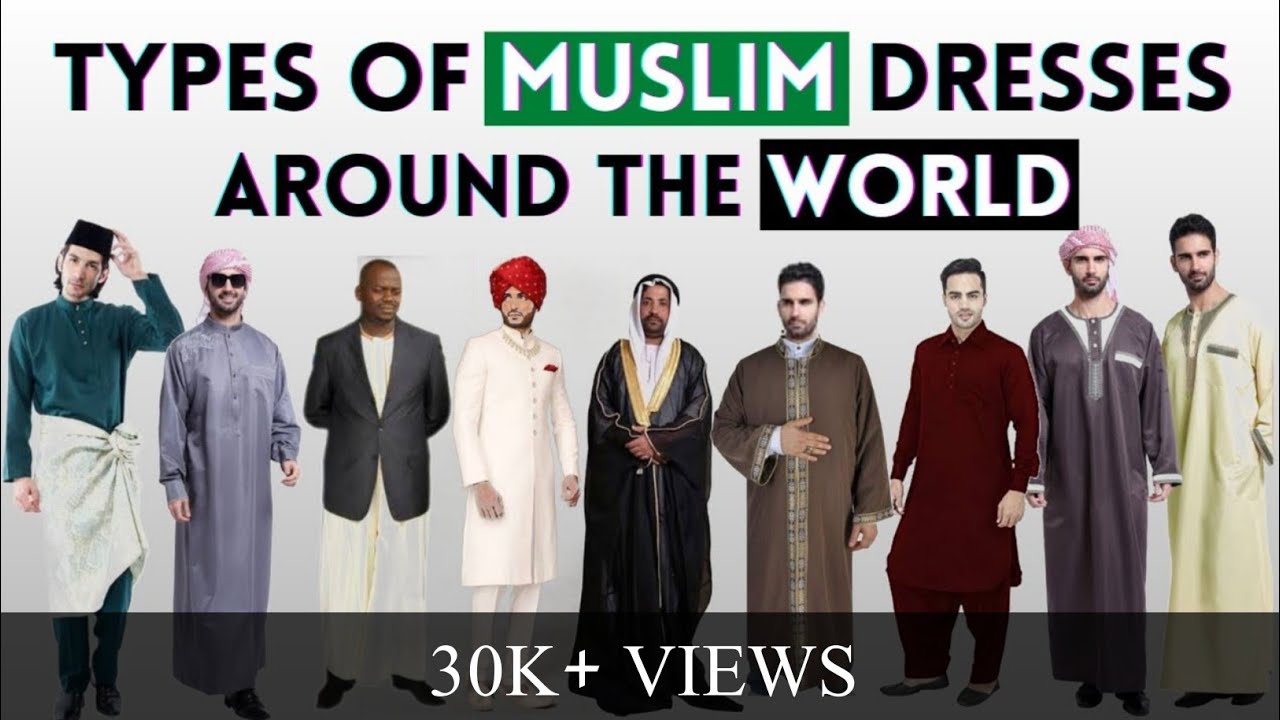The image features a visually engaging thumbnail, seemingly designed for a YouTube or social media video titled "Types of Muslim Dresses Around the World." The title is prominently displayed at the top in bold black font, with 'Muslim' highlighted in white text within a green rectangle, and 'World' highlighted in white text within a black rectangle. Below the title, there is a lineup of nine men of varying ethnicities, each showcasing different types of Muslim attire. The garments range widely in style and color, from traditional robes and turbans to modern suits, including shades of white, cream, yellow, purple, pink, teal, red, black, brown, and burgundy. At the bottom of the image, a gray banner reads "30K plus views" in white capital letters. The men are positioned against a flat gray background, standing in a line and facing the camera, offering a diverse representation of global Muslim dress styles.